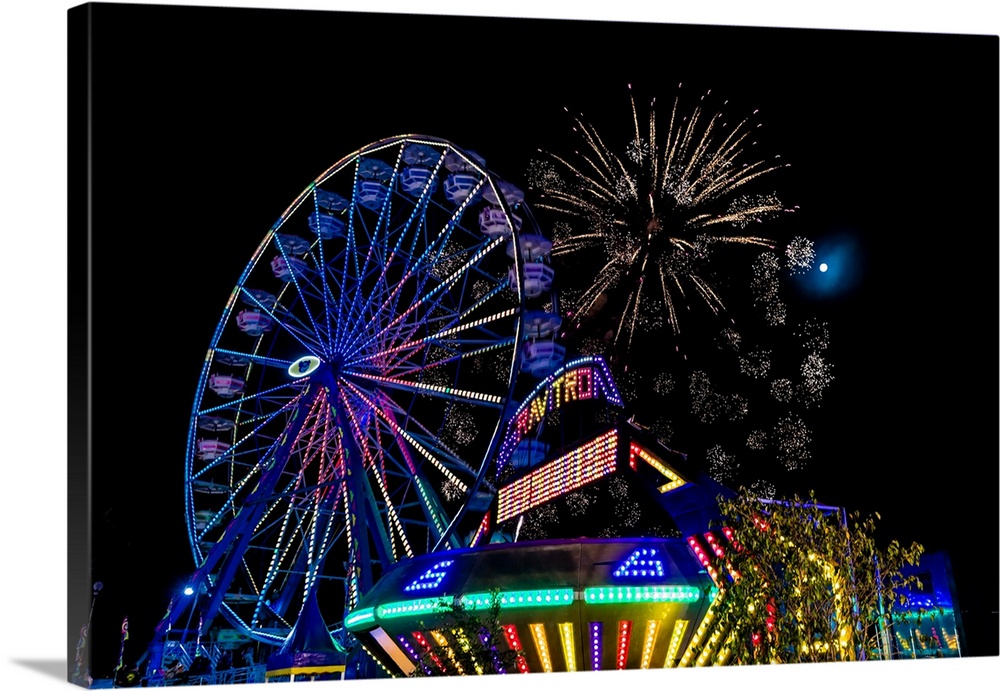This is a highly detailed photograph printed on canvas depicting a bustling carnival scene at night. The central focus is a large Ferris wheel adorned with neon lights in colors fading from blue to reddish-yellow along its spokes. Surrounding the wheel are various carnival rides and attractions, including the distinct Gravitron with its archway lit up in vibrant blue neon lights. The dark night sky is dramatically illuminated by colorful fireworks in the distance, with a hint of a glowing blue moon adding to the scene's magical ambiance. The multitude of neon lights in colors such as purple, pink, white, green, and yellow bathes the entire carnival in a mesmerizing glow, highlighting the structures and few trees that are part of the setting. The highly realistic image does not show any motion, capturing a still, vibrant moment of the festivities.